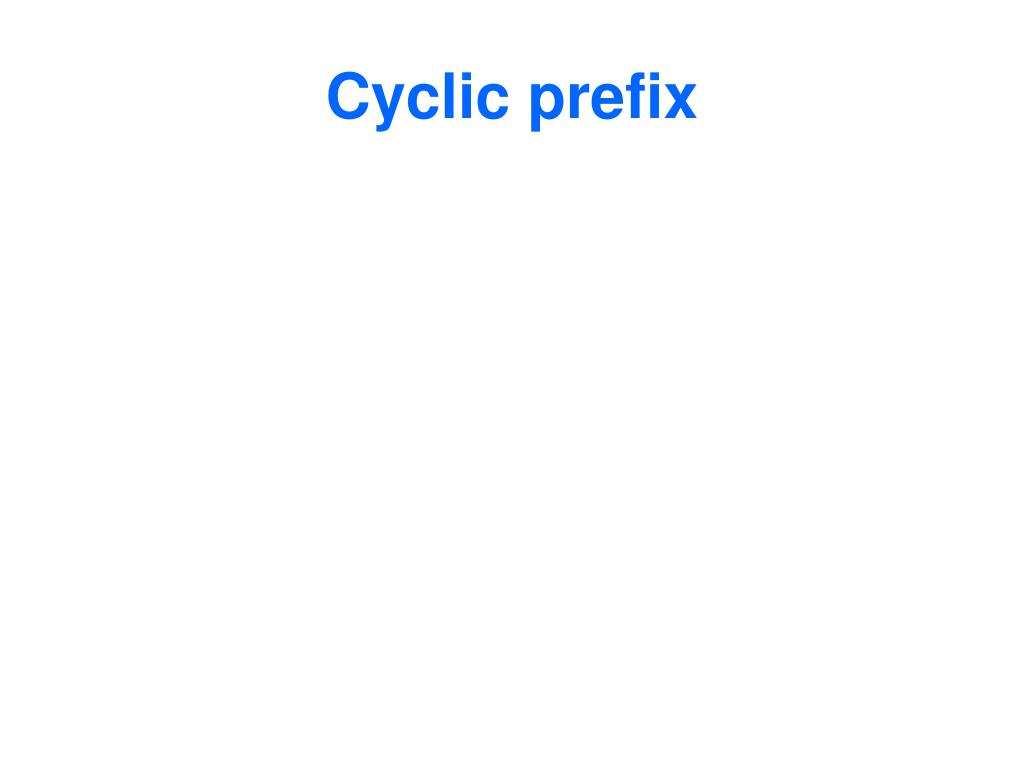The image features an entirely white background that blends seamlessly without any borders or edges. Positioned near the top, about seven-eighths of the way up from the bottom and not centered in the middle, are the words "cyclic prefix." These words are written in a non-fancy, bluish-purple, Smurf-blue text. The first word is capitalized ("Cyclic") and the second word is not capitalized ("prefix"). There are no other objects, markings, or additional text present in the image.